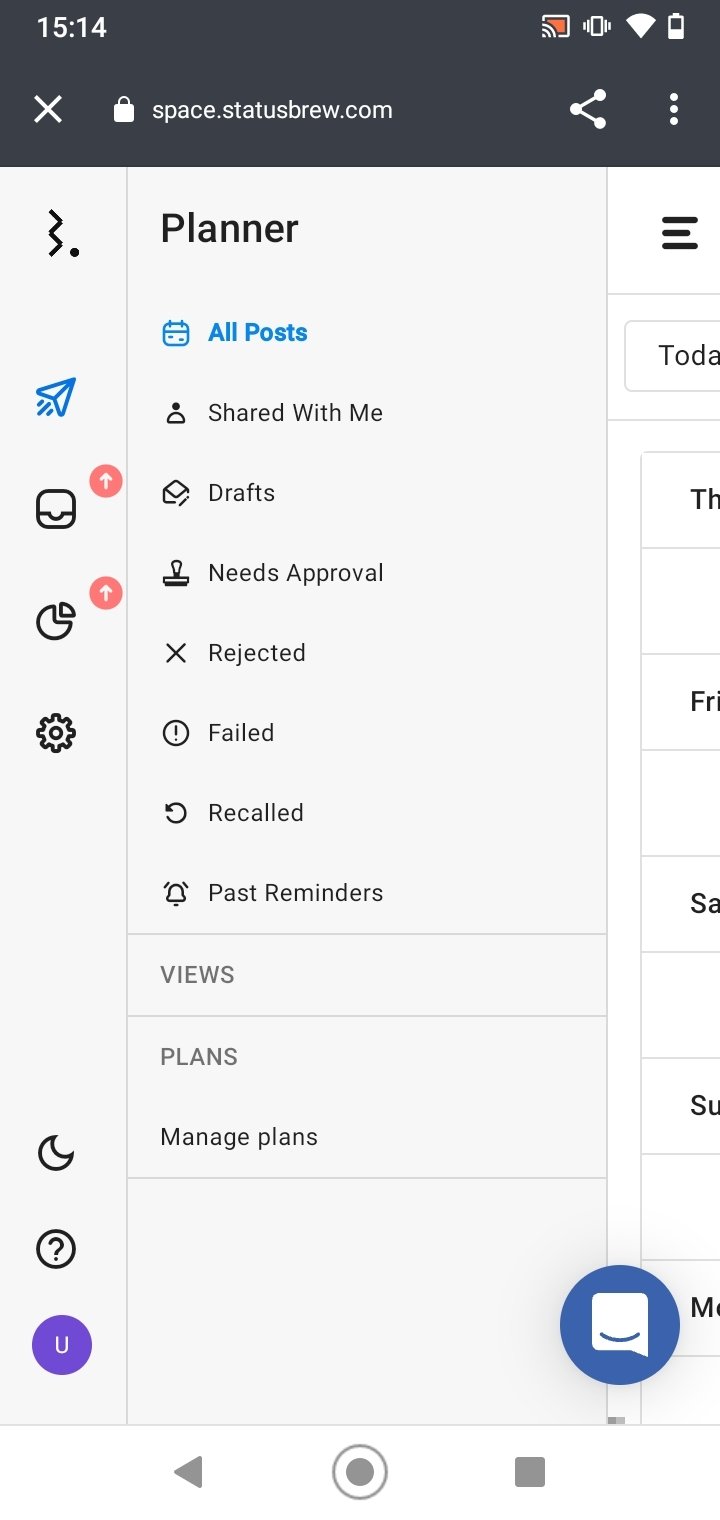This image is a screenshot of a smartphone displaying a web interface for a planning application, specifically on the site "space.statusbrew.com."

The top of the screen features a gray status bar with various elements in white. In the upper left corner, the time is displayed as "15:14." Adjacent to it, there are icons indicating battery status, Wi-Fi connectivity, and two additional, unrecognized icons. Also within this top section is a share button.

Centrally located on this bar is a search field containing the URL "space.statusbrew.com." Beneath this, the main interface features a white background. The word "Planner" is prominently displayed in black text, followed by a blue-highlighted "All Posts."

Below this heading, a columnar list in black text includes the following categories: "Shared with me," "Drafts," "Needs approval," "Rejected," "Failed," "Recalled," and "Past reminders." To the left of these categories are four icons: one resembling a share icon, another possibly for uploading images, a third that looks like a pie chart, and a fourth that appears to be a settings option.

Further down, there are mentions of three additional lists— "Views," "Plans," and "Manage Plans"— though specific details are not shown in the screenshot. Flanking these lists are three icons: a crescent moon, a circle with a question mark, and a purple circle with a white "U" inside.

In the lower right corner of the screen, there is a blue circular button with a white square in its center. At the very bottom of the screen, navigation buttons include a back button, a home button, and an overview (square) button.